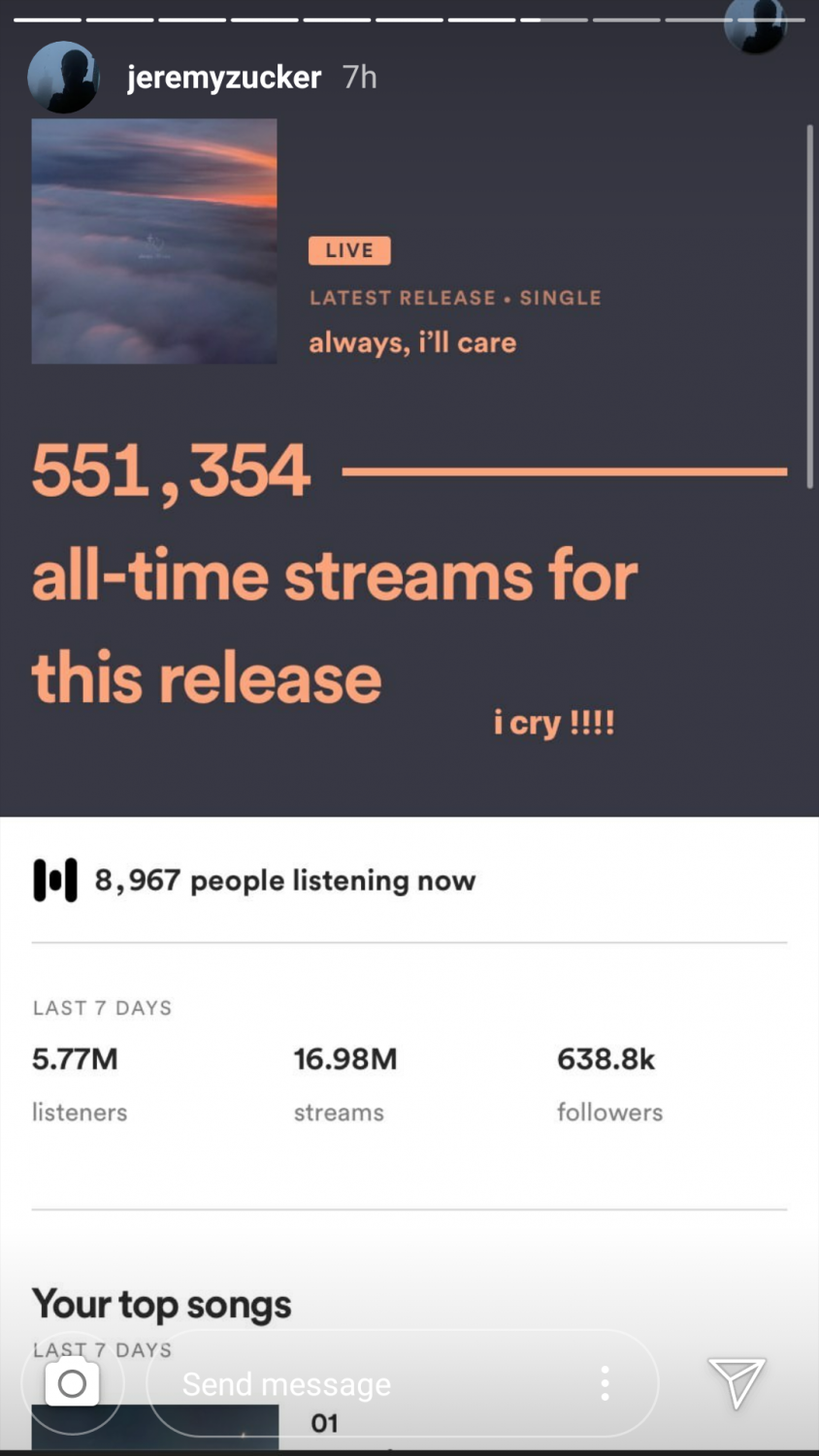The image features a predominantly gray square at the top. At the very peak of the square, there's a series of dashed white lines transitioning into gray lines towards the right. Positioned within and below these lines are circles containing a silhouette of a head. Beneath the lines, the circle is labeled with "Jeremy Zucker 7H."

The main part of the image showcases a visually ambiguous scene that could be either a sunrise or sunset. Overlaid on this scene is an orange rectangle labeled "Live." Directly below it reads: "Latest Release: Single - Always, I'll Care." 

Additionally, the numbers "551,354" appear, followed by the phrase "All times dreams for this release" in an orange line. Towards the right side of the image is the text "I cry!!!!" with four exclamation points for emphasis.

The bottom section of the image features a gradient square transitioning from white at the top to gray at the bottom. This section includes two long black lines with a shorter black line nestled between them. The text here states "8,967 people listening now."

A gray line separates this from another set of statistics: "Last 7 days: 5.77M listeners, 16.98M streams, 638.8K followers." Another gray line divides this from a new section titled "Your top songs last seven days" which includes an icon of a camera and the text "Send Message" next to it. To the far right, there’s a vertical stack of three dots, an icon resembling a paper airplane, a gray or black rectangle, and a black line at the bottom.